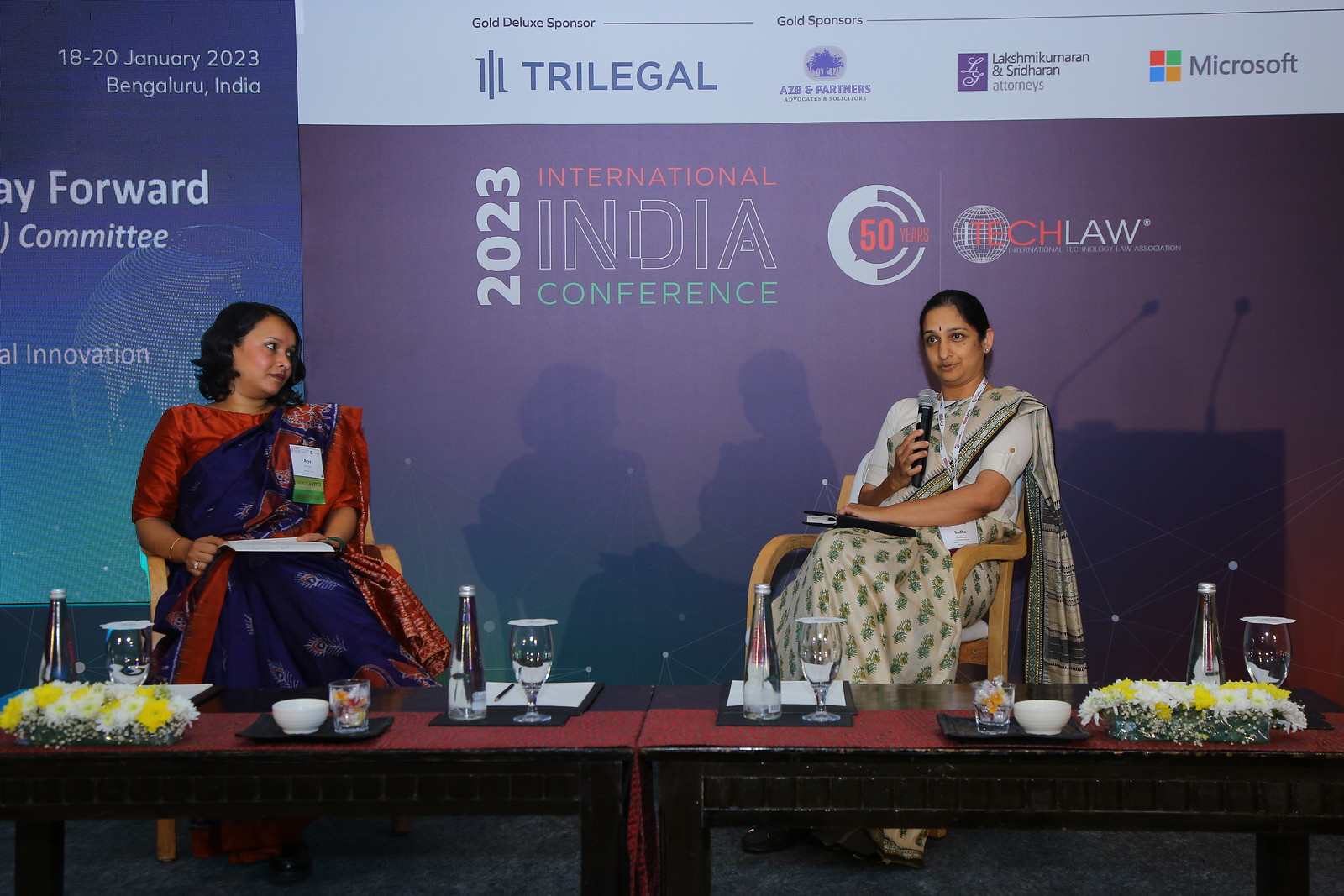This rectangular photograph, taken at the 2023 International India Conference, captures two women seated on a stage panel against a detailed backdrop. The backdrop prominently features the conference title, "2023 International India Conference," along with an array of sponsor logos including Trilegal, AZB and Partners, Microsoft, and Lakshmikumaran & Sridharan Attorneys. To the left, another banner in blue with white type reads "18 to 20 January 2023 Bengaluru India Forward Committee Innovation," although the beginning of the last word is cut off. 

In front of the backdrop, the two women are sitting in chairs behind a set of pushed-together tables, adorned with fresh yellow and white flowers, small white bowls, glasses, both short and tall, and glass bottles of water. The table setup also features a red or burgundy table runner down the center. The woman on the left, dressed in an ornate orange and bright purple sari, holds a book and gazes towards the woman on the right. The woman on the right, wearing a predominantly beige and plaid dark gray sari, is speaking into a microphone, presumably addressing the audience. Both women, with dark skin and black hair, are enveloped in traditional Indian attire, contributing to the cultural richness of the scene.